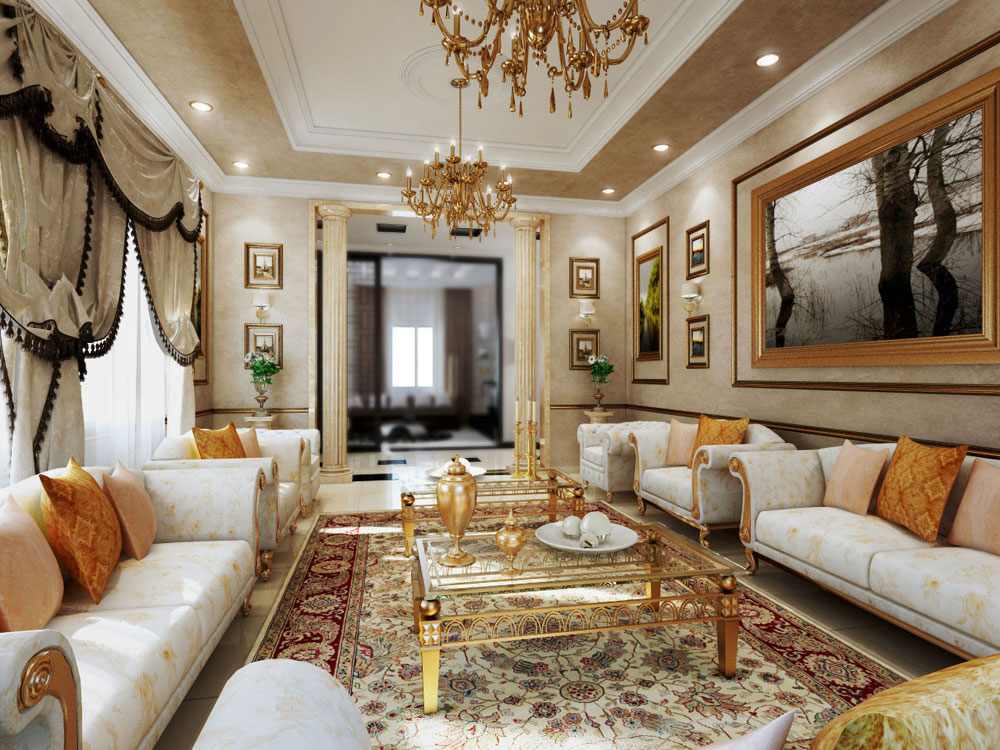The image showcases an opulent and spacious living room, characterized by its luxurious decor and abundant gold accents. The white ceiling, bordered in the same color, features two elaborate gold chandeliers adorned with beading and candle-style lights. The walls are adorned with several framed artworks, including a prominent black-and-white landscape portrait and other still images, adding a sophisticated touch.

Below the artwork, four cream-colored sofas with orange and gold throw pillows provide ample seating, arranged symmetrically around an elegant central area. Two gold-trimmed coffee tables with glass tops sit on a large, ornate Persian rug. The tables are decorated with items such as a candelabra, a tray with spherical objects, and a gold chalice-like container. 

On the far side of the room, a large window with tan and brown-trimmed curtains allows natural light to filter in, complementing the cozy yet grand atmosphere. Decorative elements like green plants in flower pots further enhance the room's inviting, lush aesthetic. The overall ambiance of the room is one of high-end elegance, blending classic luxury with modern comfort.